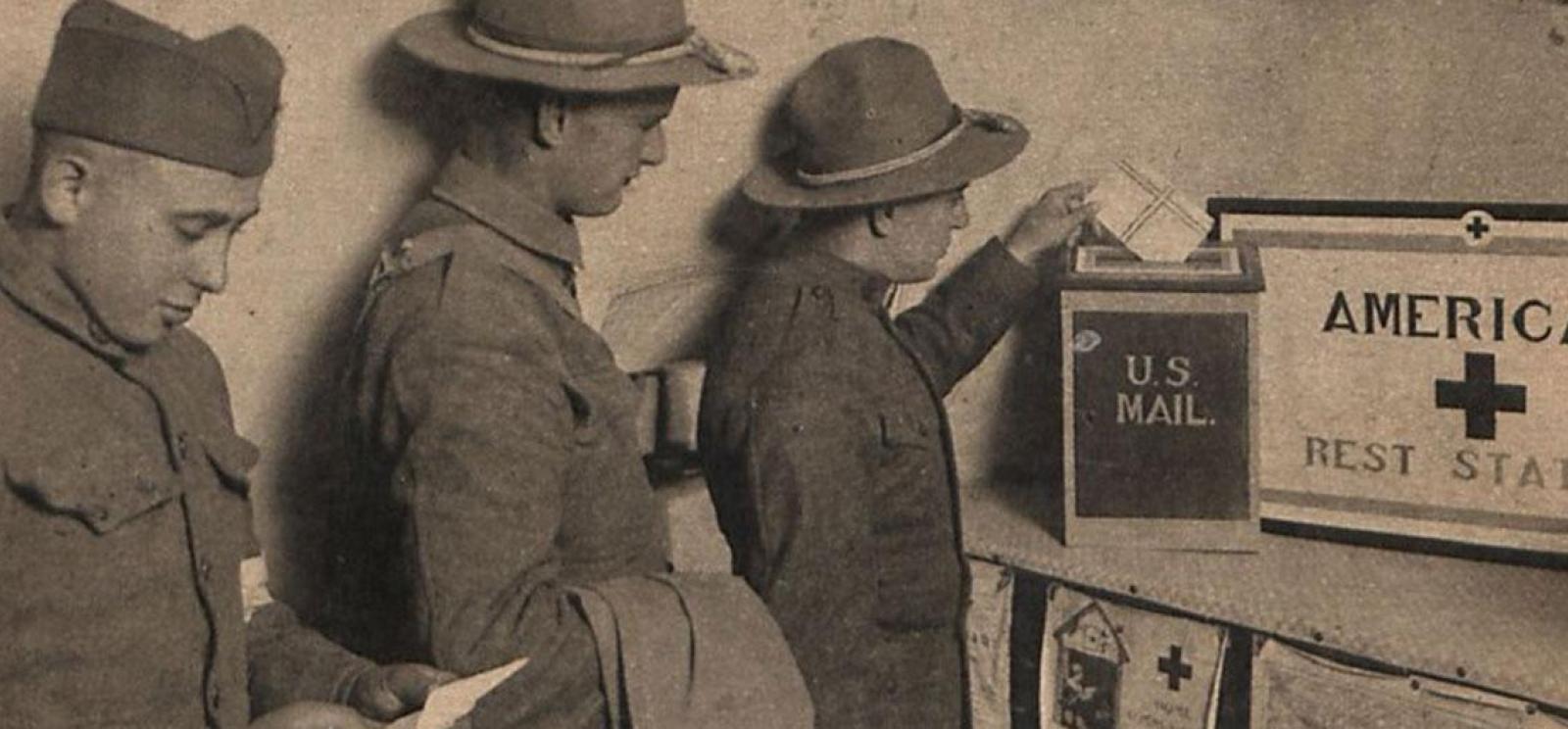This sepia-toned photograph, likely from World War I or the early 20th century, captures a moment of three soldiers in uniform at an American Red Cross rest station, possibly in France. The scene is set inside a tent, with a horizontal orientation that perfectly frames the action. The first soldier is placing a postcard or letter into a U.S. Mail box positioned on a table. The second soldier, holding a jacket in his right hand, watches attentively. The third soldier, distinguishable by his different style of hat that resembles a fedora, is engrossed in reading a letter he appears to be preparing to mail. The partially visible sign on the right reads "America Rests STAT," likely short for "Rest Station," featuring a prominent black cross in its center. This poignant image provides a glimpse into a moment of respite and connection for these servicemen during a time of conflict.